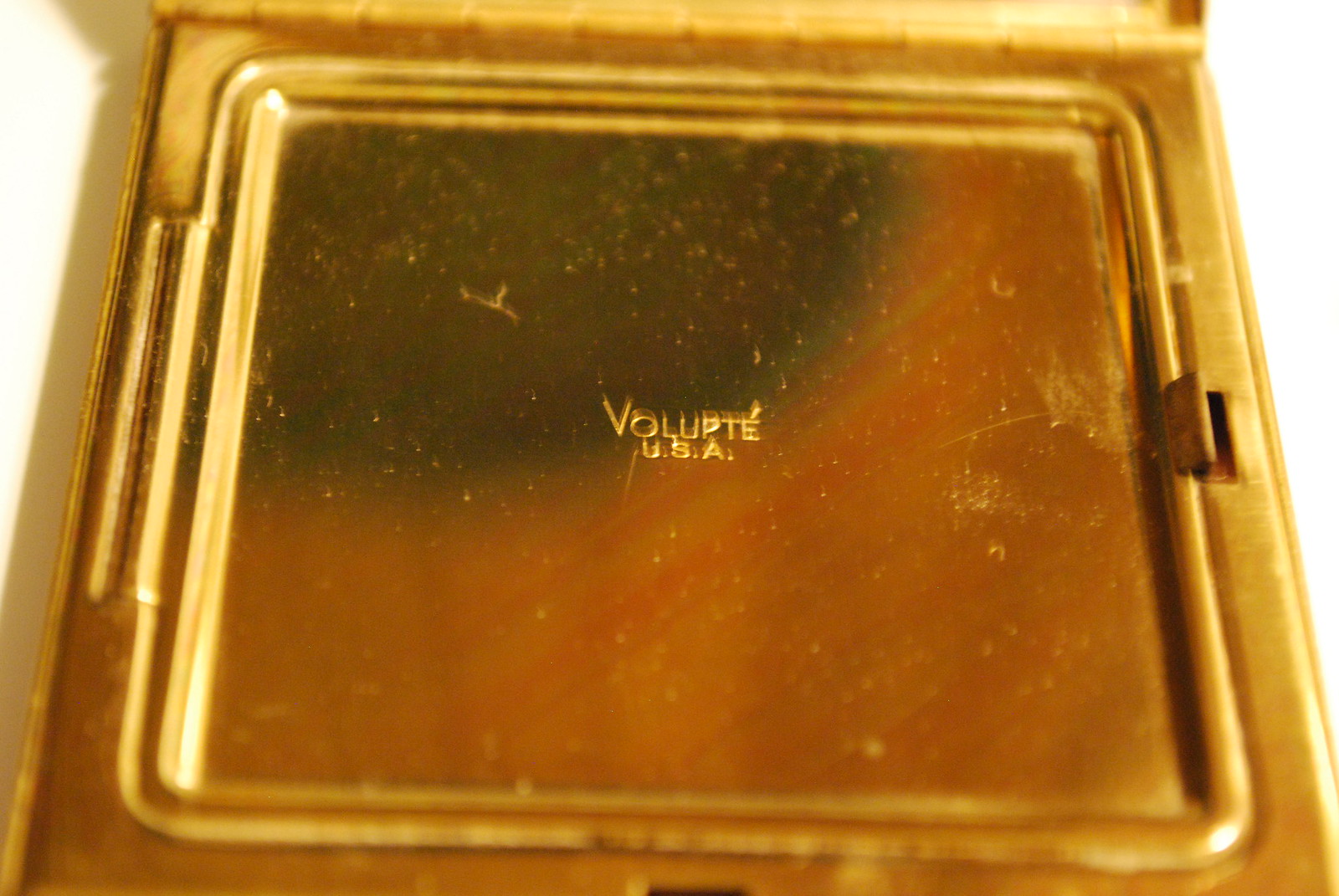The close-up color photograph features a square, brassy gold object that appears to be the underside of a compact or small box. Central to the image is embossed text: "VOLUPTEE" with an accent mark over the final 'E', and "USA" written beneath it in capital letters. The surface of this object showcases a blend of gold tones with a hint of orange, and exhibits a patina that suggests it might be metal that has aged with time. A visible seam runs around the object, and on the right side, there is a latch midway along the edge, hinting that this could be a lid. Additionally, a hinge on the opposite side suggests that this item can open and close, reinforcing the idea that it might be a vintage compact or a similar hinged container.